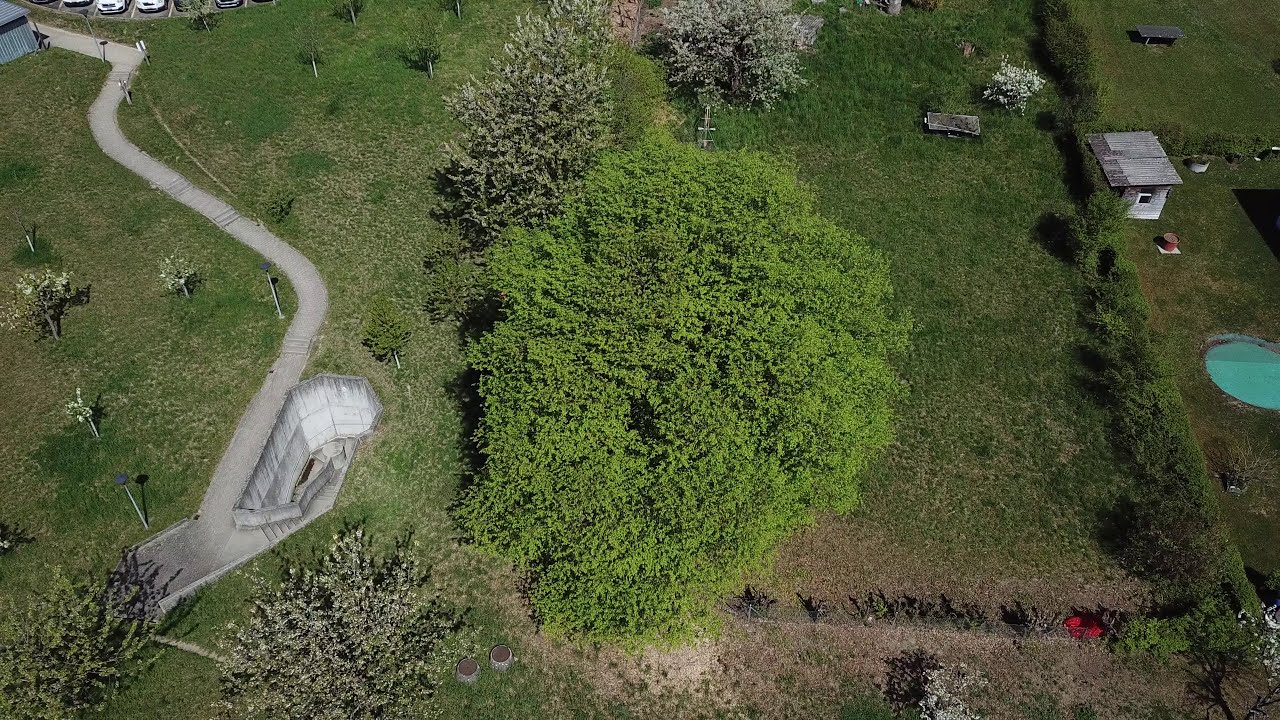The aerial photograph showcases a rural landscape featuring extensive green grasslands and various trees. Dominating the center of the image, a substantial tree is surrounded by a few smaller trees. A cement walking path, starting at the upper left-hand corner, meanders through the image in a winding pattern before ending at the lower left corner near a structure, possibly a wall. On the right side of the image, a vertical hedge separates two parcels of land—on one side, predominantly open grass with trees, and on the other side, a small shed and what appears to be an above-ground swimming pool. The image cuts off at the right edge, partially obscuring the pool and shed.